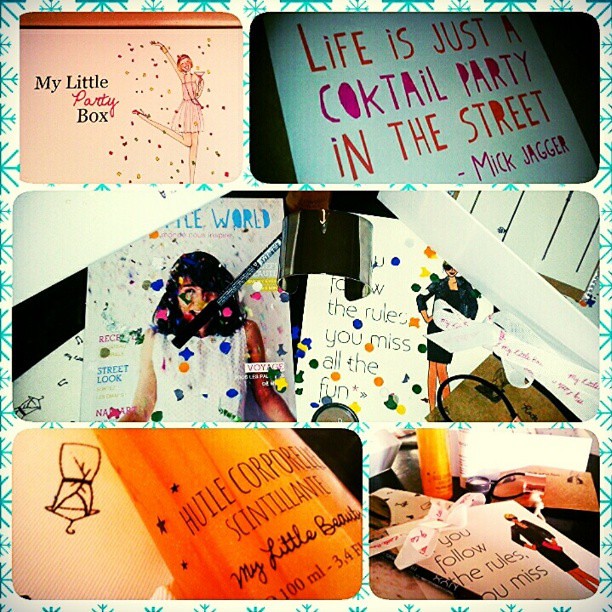This is a photo collage with a white background adorned with blue snowflakes and various teal and diagonal line embellishments. The collage consists of five images arranged in a roughly vertical rectangular layout: two images on the top row, one in the center, and two on the bottom row. 

The top left image is predominantly pink and features black writing. It depicts a woman with her right arm raised, her right leg kicked out, seemingly holding a drink, wearing a dress with a necklace, and tossing confetti. The text reads "My Little Party Box," with "Party" highlighted in red.

The top right image has a black background with a white piece of paper and text in pink and orange letters that quotes Mick Jagger: "Life is just a cocktail party in the street."

The central image appears to be an assortment of magazines, markers or eye pencils, and jewelry scattered on a table. Visible elements include a magazine with a woman in a white shirt amidst confetti, a silver cuff bracelet, a magazine or photo with the text "You miss all the fun" featuring a woman in a black dress, among other unreadable papers.

The bottom left image likely depicts a drawing of a dress on a hanger next to an object labeled "Huel Corporel Cintilante, my little beauty," suggesting it might be a body spray.

The bottom right image provides a wider view of some of the items from the central image, including the body spray, the magazine or photo with the "You miss all the fun" message, a hair tie or scrunchie, a ribbon, and what is confirmed to be an NYX eye pencil.